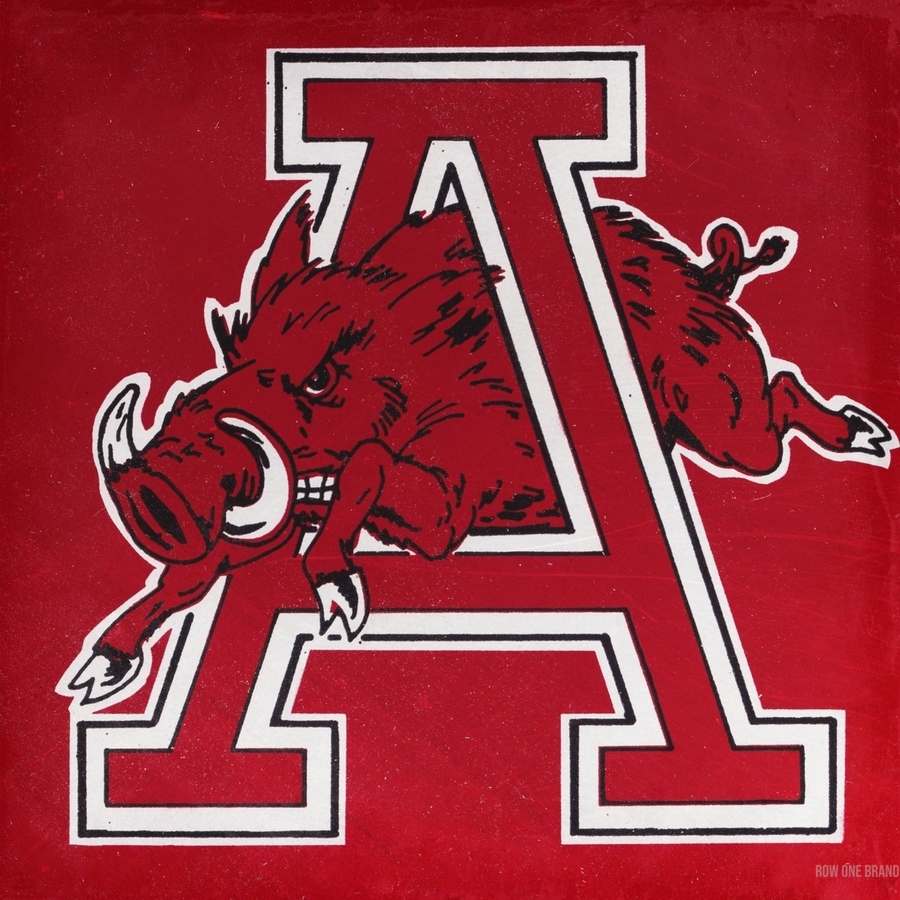A detailed poster for a sports team features a deep red square background. Dominating the center is a bold, block letter "A" with multiple layers: an outer white border, followed by a black line, another white space, and a black-lined inner edge, all enclosing the red "A". A fierce, red pig-like animal with white tusks protrudes from the center of the letter. This boar-like creature has a snarling mouth displaying white teeth and intensely staring black and white eyes. Its body is red with black splotches, black and white hooves, and a matching tail with black lines. The entire animal figure is accented with a white embossed outline, providing a strong, standout appearance. In the bottom right corner, the caption "ROW ONE BRAND" is elegantly written in gray capital letters, completing the design.